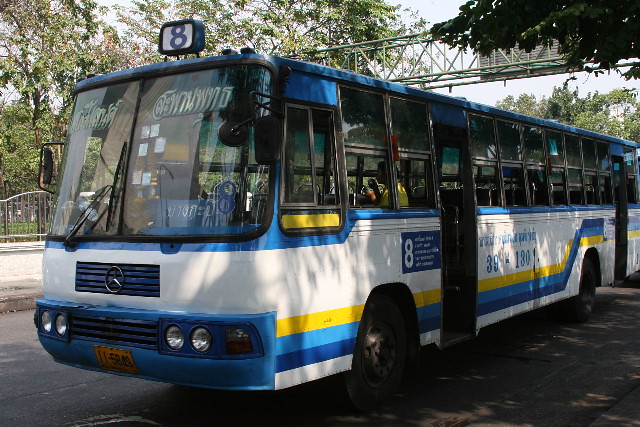In this daytime photograph, a large blue bus prominently featuring a thick white stripe in the center is captured against a backdrop of surrounding trees, suggesting a park-like setting. Accentuated with additional stripes of yellow, light blue, and dark blue spanning from the front grill to the back, the vehicle showcases the logo of Mercedes-Benz on its front. Thai letters adorn the bus, identifying it as a vehicle from Thailand, with the number "8" displayed on the top and sides. The serial number "39180" is also visible along with more Thai script. The bus has tinted windows and its doors appear slightly ajar, indicating it is parked. Inside, a single person is seated towards the front, facing away from the camera and possibly applying makeup while wearing a yellow shirt. This individual might be the driver, as there are no other passengers visible inside. In the distant background, a bridge can also be seen, adding depth to the scenic setting.